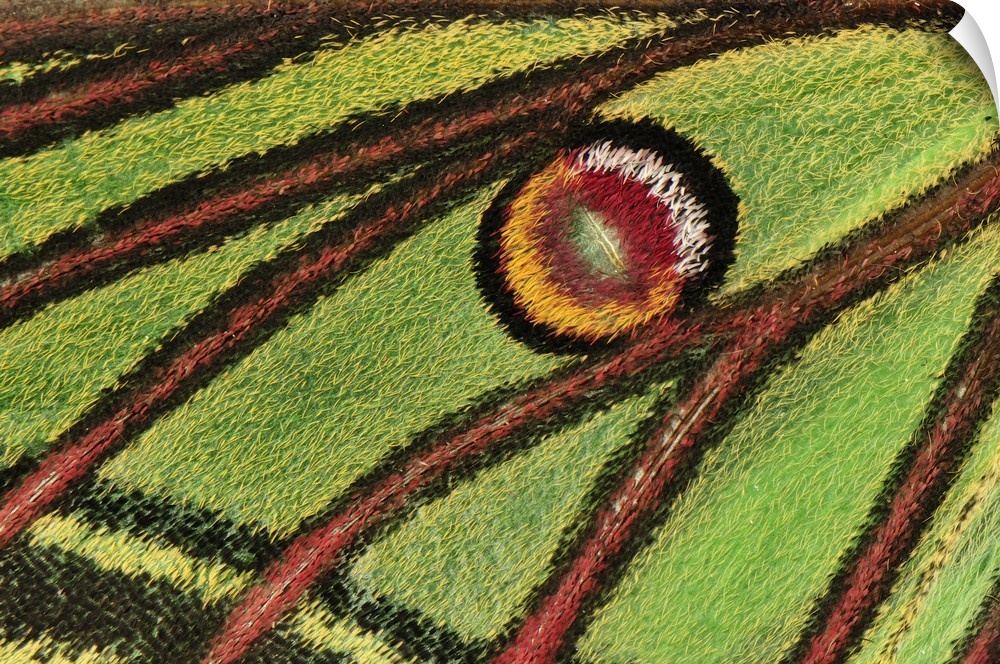This digital mock-up depicts an abstract art piece resembling a fibrous rug or textured canvas print, characterized by intricate, vein-like patterns. Dominating the image is a central motif that appears to be an eye. This eye features a multi-layered design: a black border, followed by a concentric yellow and white layer, and a vibrant red and orange core. Surrounding the "eye" are red veins outlined in black, which radiate outward, creating a sense of movement across the piece. These veins contrast strikingly with the green rug material or background, which fills the spaces in between. Towards the lower left corner of the composition, a sequence of alternating yellow and black stripes is visible. Additionally, in the top right corner, a folded segment reveals a white background, suggesting a three-dimensional aspect or a paper-like division. The entire depiction hints at a close-up view of a Spanish moon moth wing, with brown twig-like lines extending from the right to the left across the green backdrop, further enriching this abstract and visually dynamic representation.